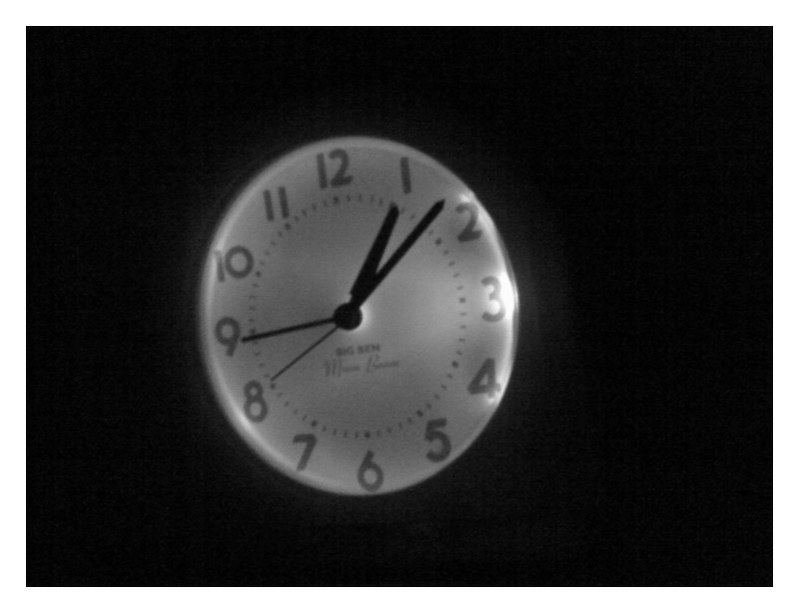This image features a detailed depiction of a round clock face set against an entirely black, noisy background. The clock appears to be floating slightly left of center, and it has a somewhat blurry, illustrative quality, possibly created using a graphics program like Photoshop. The clock's surface looks metallic and highlights are visible around the numeral three. The face itself is white with dark gray numbers lined meticulously in a block style. Surrounding the numbers, minute-indicating lines are also visible. There are four hands on the clock – a black minute hand, hour hand, second hand, and an additional wider hand about the same size as the hour hand. The time displayed is approximately 1:12. Centrally located beneath where the hands meet, there is black text; part of it reads "Big Ben," though the rest is illegible. The intricate details and blend of textural shadows give the clock a unique visual appeal.